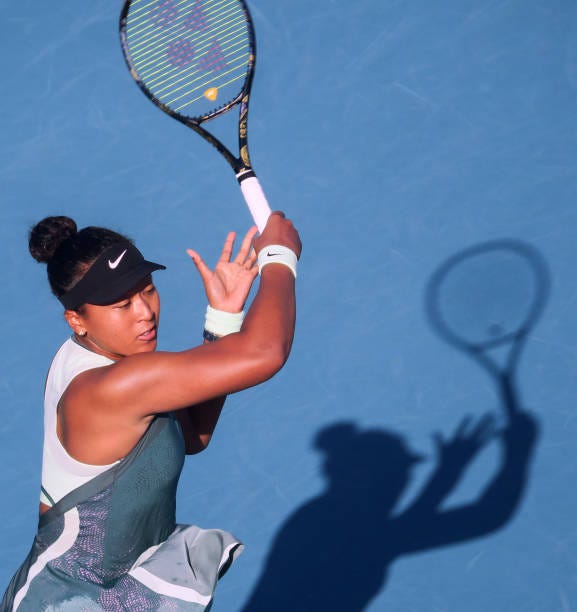In this photo, a young, serious-looking Asian woman is playing tennis, set against a solid medium blue background. Her dark hair is neatly pulled up into a bun, and she wears a black Nike visor. The woman is dressed in a sleeveless white top layered with a gray mesh outfit that includes a distinctive white stripe down the side. Matching white wristbands with the Nike emblem accentuate her muscular arms. She grips a black tennis racket with a white handle and green strings, lifting it with one hand while the other provides support. Her focused expression and determined stance cast a sharp shadow of herself and her racket against the blue backdrop.